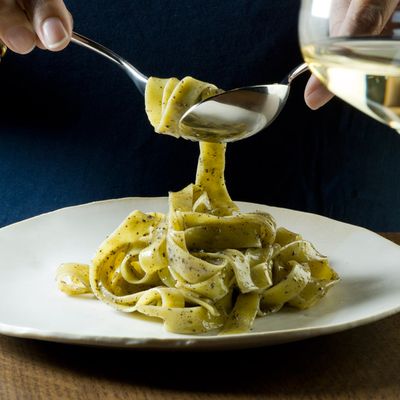The image captures a close-up view of a white plate filled with yellow fettuccine Alfredo on a brown wooden table. At the top left corner of the image, a hand is seen holding a fork that has spiraled some pasta noodles, while another hand at the top right steadies the pasta with a spoon. The background features a dark blue cloth, possibly the shirt of the person holding the utensils, adding depth to the scene. A reflective surface in the top right hints at a wine glass that is half-full of white wine, adding a touch of elegance to the setting. The overall composition presents a meticulous moment of dining, emphasizing the rich texture and color of the freshly prepared fettuccine Alfredo.